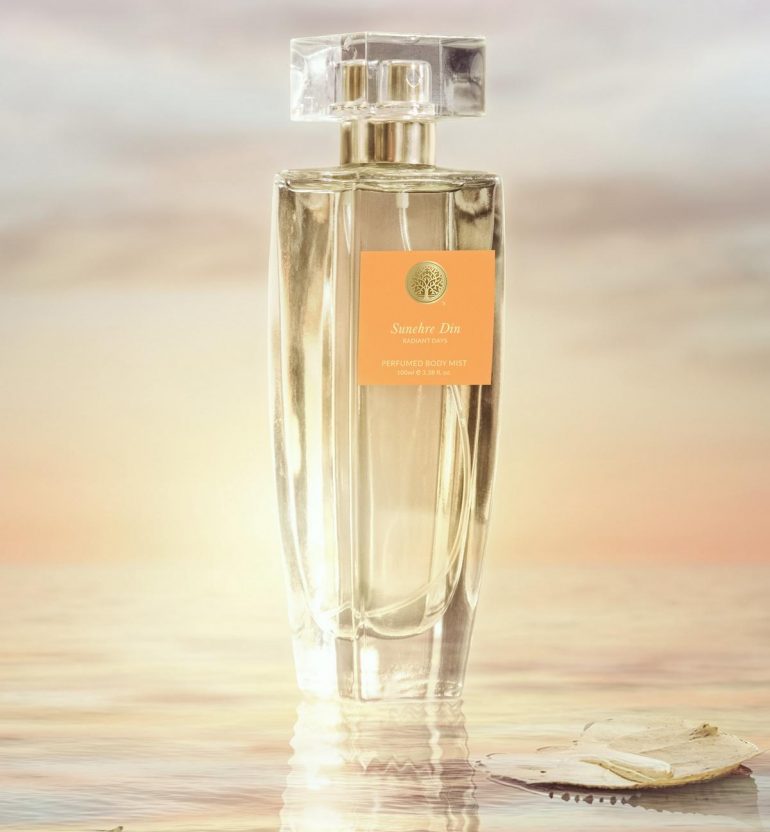This advertisement showcases a perfume bottle named "San Cher Dia," featuring a visually striking, clear glass design. The bottle has a distinctive shape, with a square form that tapers to a narrower base. It bears a delicate, peachy-orange label adorned with a light yellow script font, difficult to read but hinted to include the words "perfume" and "body mist." Prominently displayed on the label is a circular gold emblem resembling the tree of life.

Topping the bottle is an elegant, clear acrylic block, set just above a gold band, which sits on the sprayer. The perfume rests on a highly reflective surface displaying a palette of pale, dreamy colors such as yellow, peach, and pink. The background complements this ethereal setting with soft, diffuse hues of brown, yellow, and orange, evoking a serene, daybreak atmosphere reminiscent of a calm seascape, enhanced by gentle, water-like reflections and horizon-like depth.